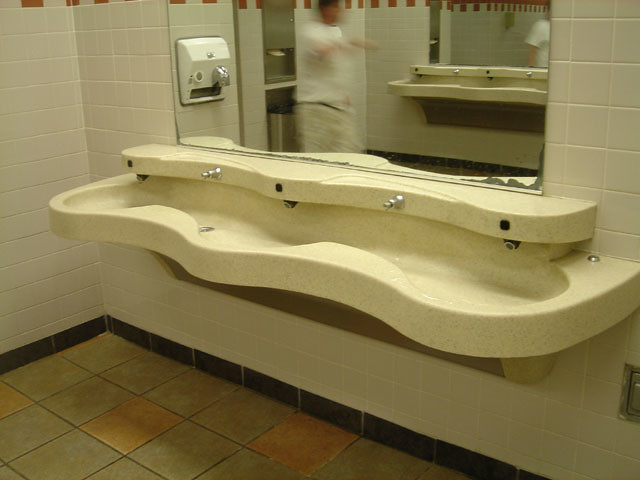This photograph captures the interior of a public restroom, specifically focusing on the sink area. The bathroom features a distinct beige or tan, curvy trough sink with a wavy design, resembling an ocean wave, made from a fake stone material. This long, continuous sink accommodates three black, motion-activated water dispensers and two silver-knobbed soap dispensers positioned between each pair of water dispensers. 

Directly above the sink is a large, somewhat faded mirror with aged, peeling metallic backing, providing a glimpse of the restroom's symmetrical layout. Reflected in the mirror is an identical setup with a second trough sink and another mirror. The reflection also reveals a white hand dryer with a silver nozzle mounted on the wall and a blurry image of a person, possibly a Caucasian male in a white t-shirt and tan pants.

The restroom's walls are tiled in a cream color with white grout, and there is a black baseboard at the bottom. The floor consists of various slate-like tiles in gray and random gold tones, resembling terracotta mixed with gray-green hues. The overall ambiance suggests a functional yet worn public restroom, likely found in a high-traffic area such as a truck stop.